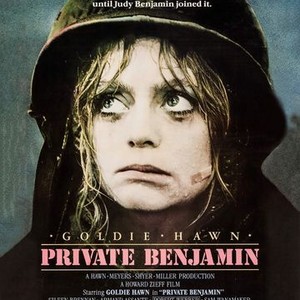This is a highly detailed movie poster for "Private Benjamin" featuring Goldie Hawn. The text at the top reads, "Until Judy Benjamin joined it," followed by "Goldie Hawn" and "Private Benjamin" written in pink text, while the rest is in white. The additional information about the movie's cast and crew is presented at the bottom. The central focus of the image is on Goldie Hawn, who portrays Judy Benjamin. She is depicted wearing a dark brown military helmet and a black coat, standing against a bluish background. Her blonde hair, appearing wet and clinging to her face, combined with smeared makeup, suggests she is in a rain-soaked setting. Her expression, looking up into the sky with sad, tired eyes, highlights a poignant moment in the film.